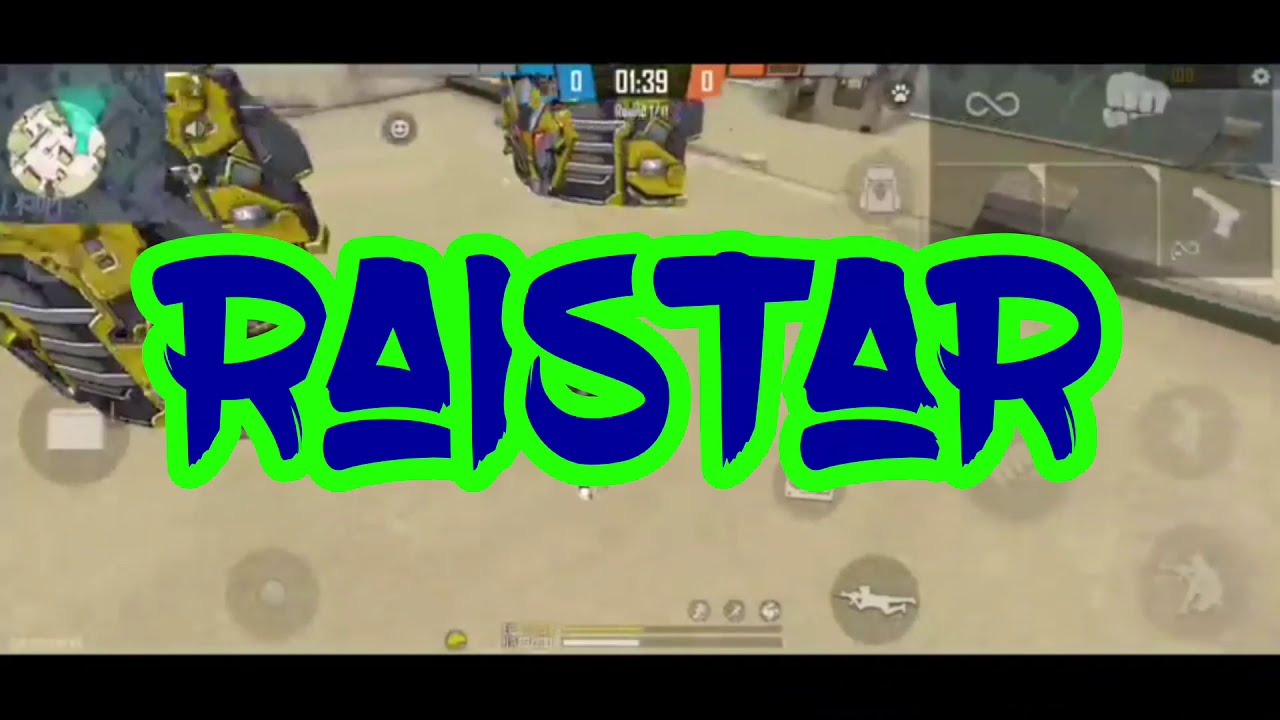The image appears to be a screenshot from a video game titled "Raystar," prominently displayed in stylized blue letters with a lime green outline across the middle. The scene likely depicts a supply room filled with military gear. In the lower portion, there's a machine gun icon, while the upper section features a timer displaying 1:39, flanked by scores of zero in both a blue and an orange background. The environment includes a sandy or beige-colored floor and various indistinguishable metallic and robotic devices. In the upper left corner, a potential map is visible, and under the game's title, in the center, is a blue zero and orange zero. Off to the right side, there’s an array of icons including a handgun, a fist, and an infinity symbol, along with the image of a soldier with a rifle in the lower right corner. The background shows silhouettes of soldiers in different stances, adding to the setting's military theme.